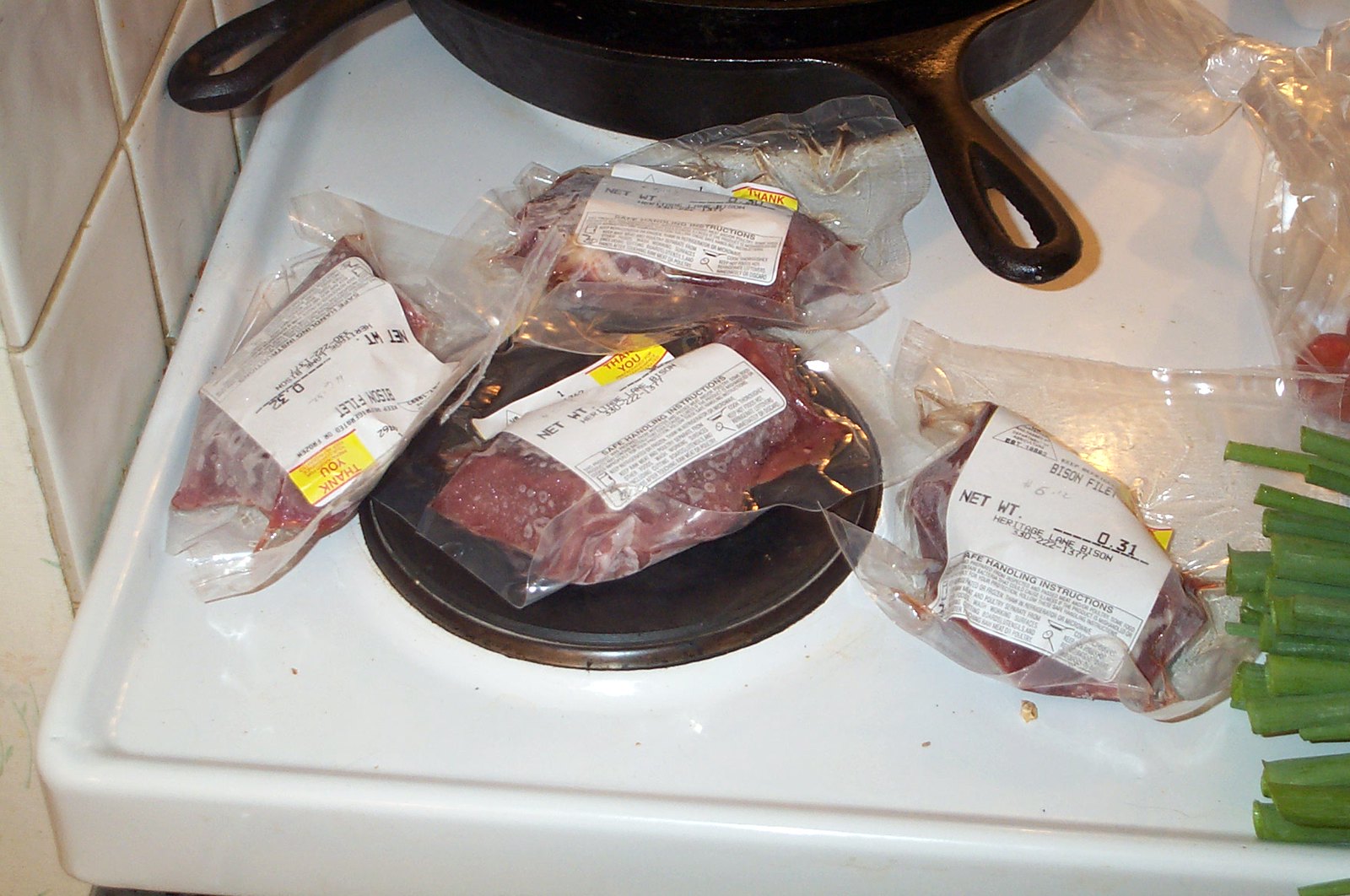This image depicts a domestic kitchen scene focused on a white stovetop adorned with various culinary items. The setting includes a bit of a light beige tiled wall on the left side. The stove itself is white with dark, discolored electric burners, and in the back, there's a cast-iron skillet, with just its handle and part of its body visible. At the forefront, there are four vacuum-sealed packages of red meat, specifically labeled as heritage land bison, each with visible weight labels. To the right, nestled on the countertop, you can see a plastic bag containing the ends of green onions and some red vegetables, possibly tomatoes. The overall arrangement suggests that the packaged meat is thawing over the stove in preparation for cooking.